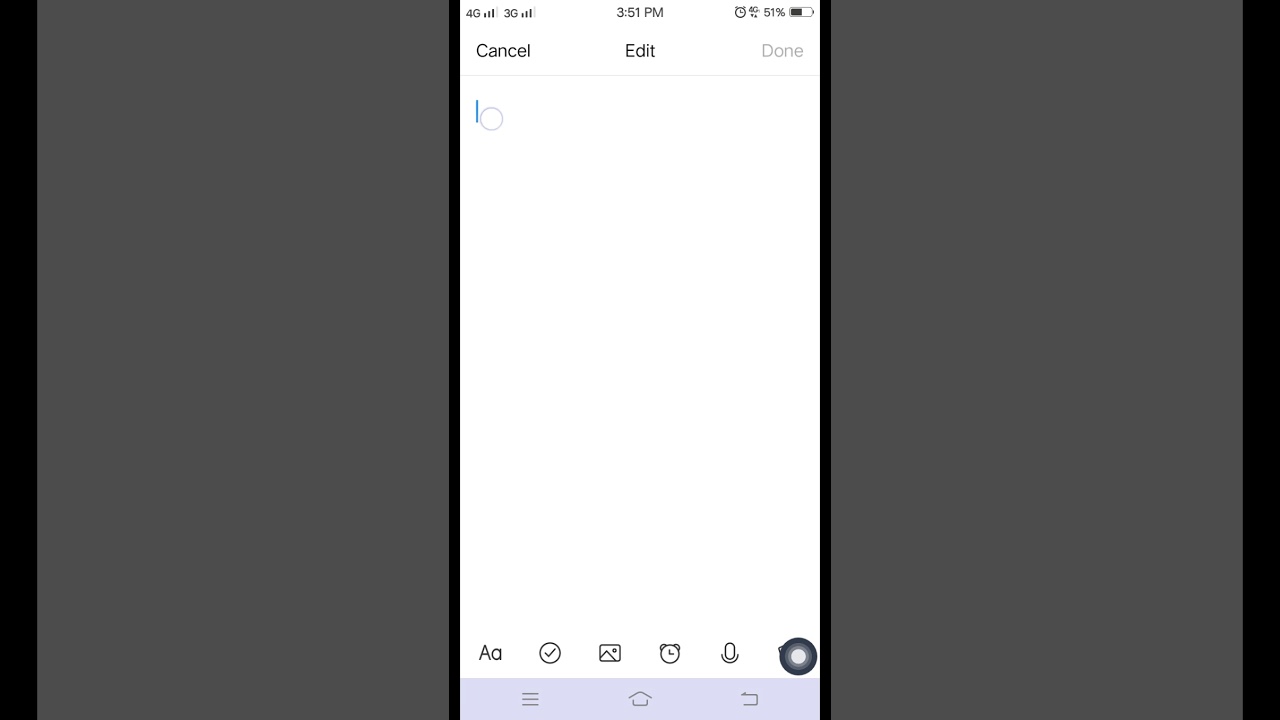A screenshot of a mobile note-taking application interface is displayed. At the top of the screen, there is an "Edit" button on the left and a "Cancel" button to its immediate left, while a "Done" button is situated on the right. Below these options lies a large, blank white page, indicating an empty note. Directly beneath the blank page is a toolbar featuring several icons: a text formatting button depicted by a capital "A" and a lowercase "a", a circled checkmark, an image icon, an alarm clock icon, and a microphone icon. The phone's standard user interface is visible at the bottom, with a menu button on the bottom left, a home button in the center, and a back button on the bottom right. The overall layout is clear and functional, designed for efficient note creation and editing on the go.